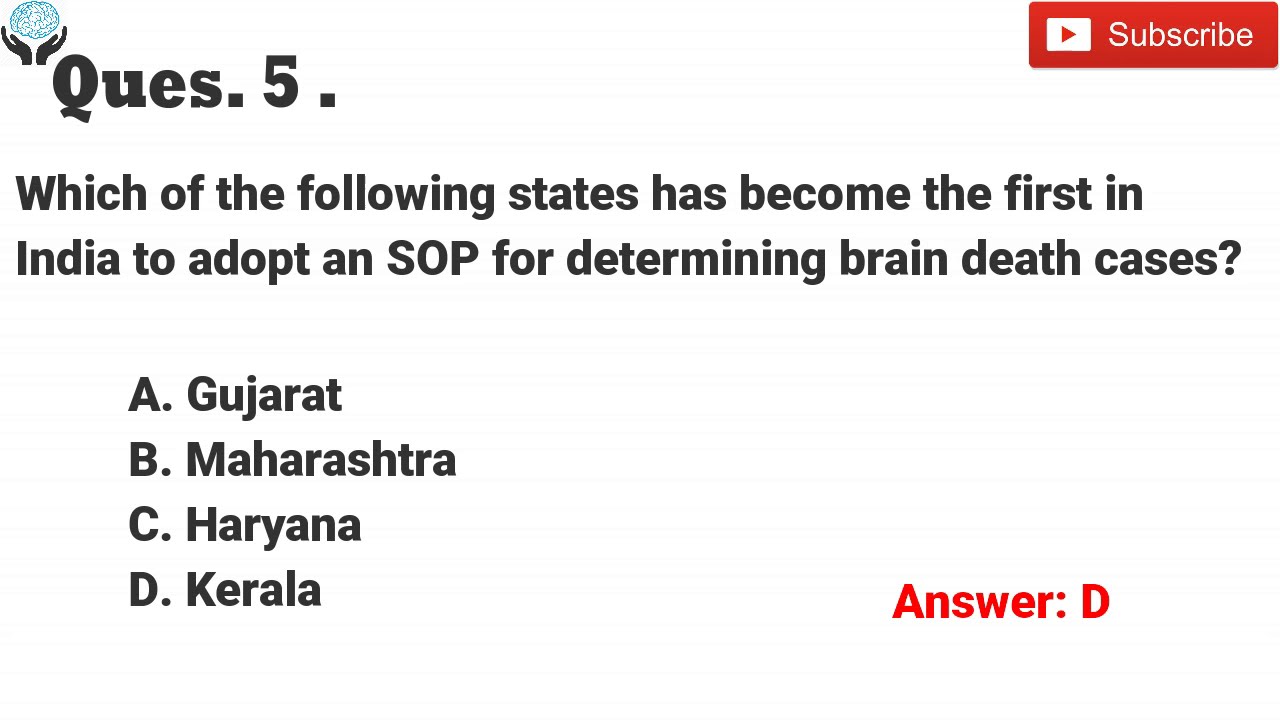The image is a screenshot of an online quiz, displayed against a mostly white background with subtle horizontal light blue lines. Centered prominently in bold black text, the question number reads "Q5." The question posed is: "Which of the following states has become the first in India to adopt an SOP for determining brain death cases?" The four answer choices are listed vertically as A. Gujarat, B. Maharashtra, C. Haryana, and D. Kerala. The correct answer, "D. Kerala," is highlighted in bold red text in the bottom right corner. The quiz interface includes additional elements: a red "Subscribe" button with white text in the upper right-hand corner, suggesting this is a video hosted on YouTube, and a logo in the top left corner showing two black hands cradling an outlined blue brain.